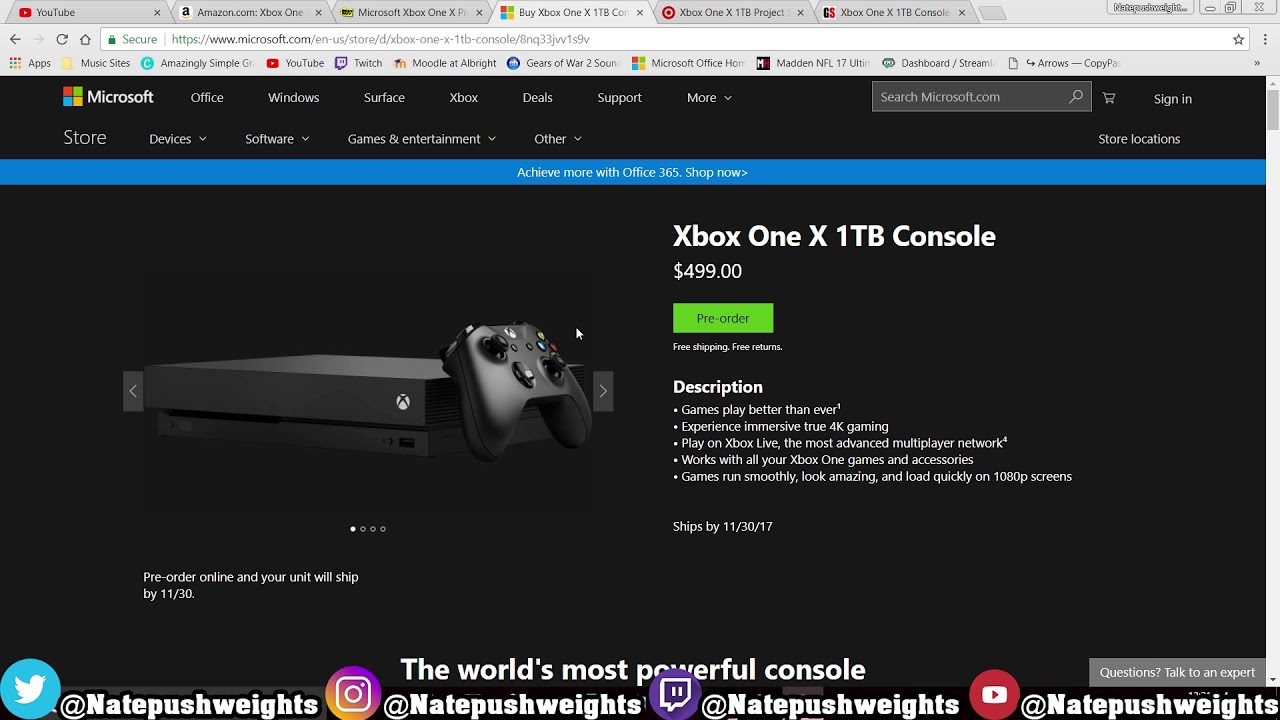The image is a horizontally rectangular screenshot taken from a computer. Along the top of the screenshot, several website tabs are visible, including YouTube, Amazon.com, Microsoft, Buy Xbox (represented by the Microsoft Store icon), Target, Xbox, and another tab with the initials "GS," which could indicate a company related to Xbox One but is not clearly identified.

Beneath the tabs, there are the standard search bar and a row of bookmarked tabs. The main content of the screenshot is centered and set against a black background, displaying the Microsoft website. The page features the Xbox One X 1TB console listed at a price of $499. A green pre-order button is positioned directly beneath the price.

Additional details on the page include free shipping and free returns. The product's description states, "Games play better than ever. Experience immersive true 4K gaming. Play on Xbox Live, the most advanced multiplayer network. Works with all your Xbox One games and accessories. Games run smoothly, look amazing, and load quickly on 1080p screens." The shipping date is noted as November 30, 2017. To the left of this information, there is an image of the Xbox console accompanied by a controller.